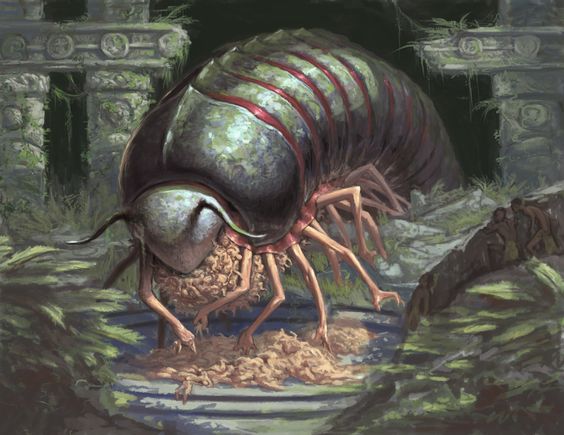The illustration depicts a surreal and unsettling fantasy scene featuring a giant, silver-colored centipede-like insect with human arms and hands in place of legs. The creature’s back is adorned with green plates, each separated by red strips, accentuating its menacing appearance. Emerging from the darkness beyond an ancient, crumbling structure that evokes the mystery of archaeological ruins, the centipede appears to be devouring a mound composed of what seems to be body parts and beige-like flesh. Flanking the scene are sporadic patches of greenery and burgeoning plants, which contrast sharply with the macabre pile of victims that the centipede grasps with its many human-like appendages. To the right of the insect, some enslaved figures seem to be directed toward the horrific heap, suggesting an offering to the monstrous entity. The overall composition of the image, slightly wider than it is tall, creates a vivid, disturbing, and fantastical narrative tableau.